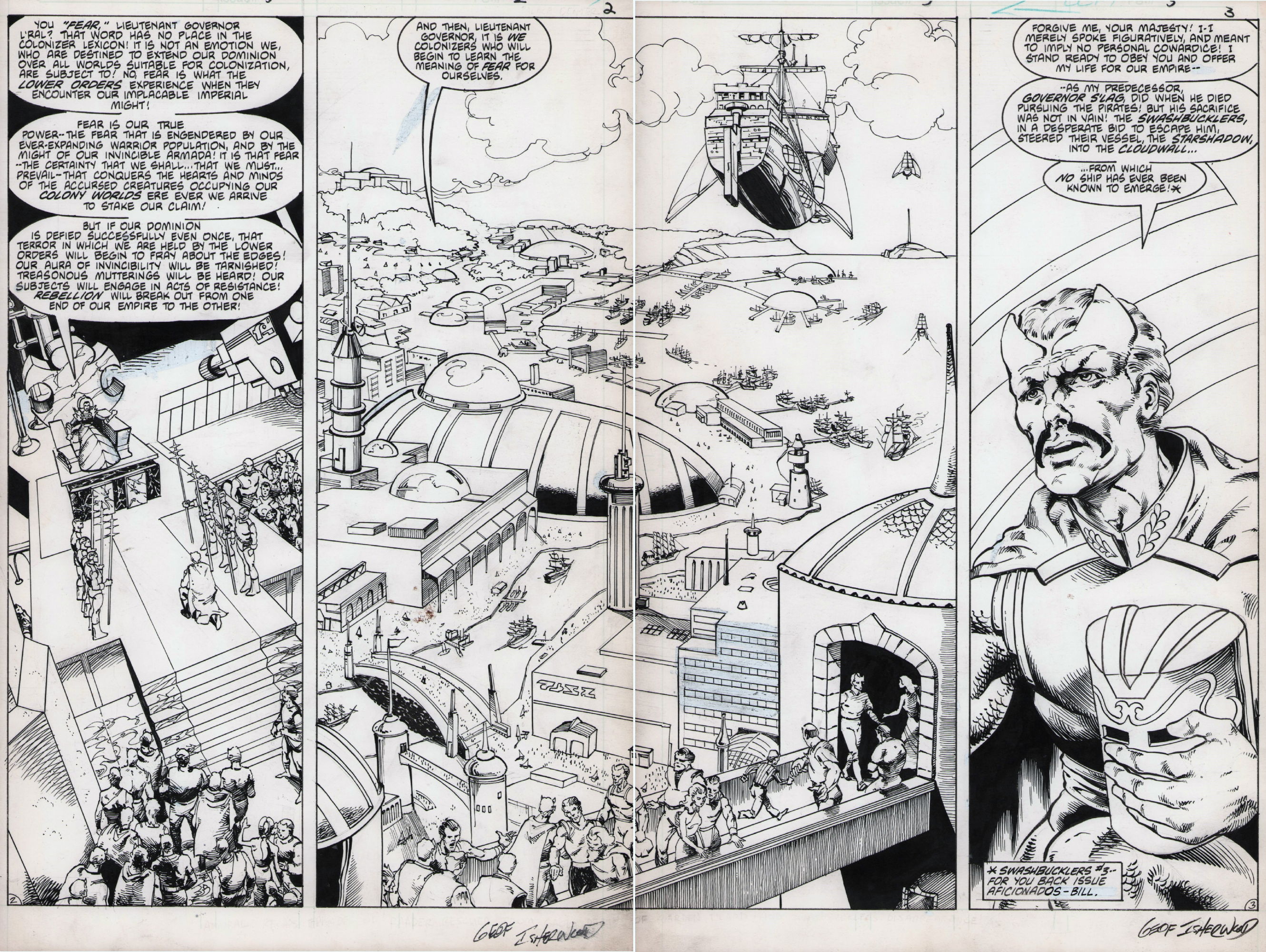This image depicts a detailed black-and-white two-page comic book spread divided into three panels. The left panel captures a dramatic top-down view of an expansive throne room. A man kneels before a figure seated on a throne, flanked by six guards wielding spears, three on each side. Behind the kneeling man are steps filled with onlookers, creating a sense of a significant event.

The middle panel, stretching across both pages, showcases an aerial view of a futuristic shoreline city. The cityscape features numerous domed buildings and piers extending into the water, with domes positioned at their ends. Boats and marinas line the shore, and a fantastical flying ship—reminiscent of an old wooden pirate vessel with wings—soars through the sky on the top right. In the foreground, people traverse a small footbridge connecting two buildings.

The rightmost panel zooms in on the kneeling man from the first panel. He is depicted holding a cylindrical, ornamented helmet and sporting a black mustache with light-colored hair. Two flat horns protrude above his eyebrows, and he wears a cloak. Although the pages are filled with text, the small font makes it difficult to discern the content. The overall style suggests a semi-realistic illustration, capturing a blend of the futuristic and the fantastical.